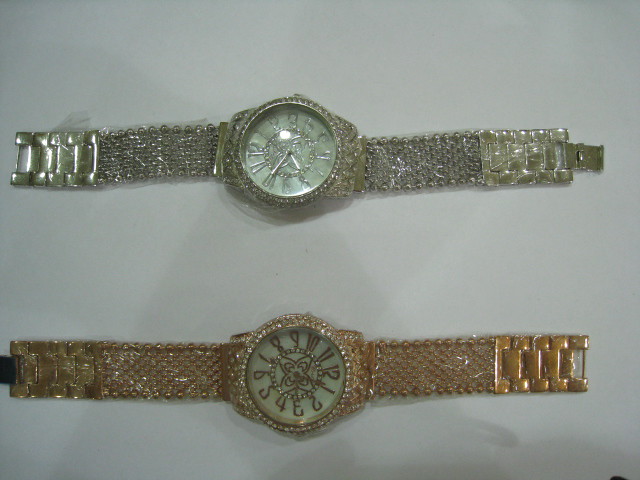The image depicts a photograph taken from above of two wristwatches positioned against a plain white background, possibly a tabletop or a piece of paper. Both watches exhibit a lavish design characterized by the extensive use of rhinestones and intricate metal ball patterns. Despite their attempt at a luxurious appearance, the watches are evidently of cheap quality. 

The watch at the top of the image appears to be silver-toned, highlighted with numerous rhinestones along the band, the rim, and the interior of the clock face. The clock face itself boasts silver numbers, silver hands, and an ornate floral design in the center. Carefully wrapped in plastic, likely to preserve their finish before being sold, the watches are displayed in an environment with minimal lighting, casting a shadow of a phone over them and creating a dim overall photo.

The second watch shown below mirrors the first in design but with a slight variation in color, described alternately as rose gold or an orange copper tone. This watch also features rose gold or orange copper-colored numbers and hands, complemented by a matching ornate floral design at its center. Both watches have similarities in their decorative elements, including chains with ball edges, adding to their ornamental appearance while indicating a lower craftsmanship quality.

A notable detail is the bright spot of reflected light on the glass of one of the watches, contrasting with the otherwise shadowy and dark composition of the photograph.